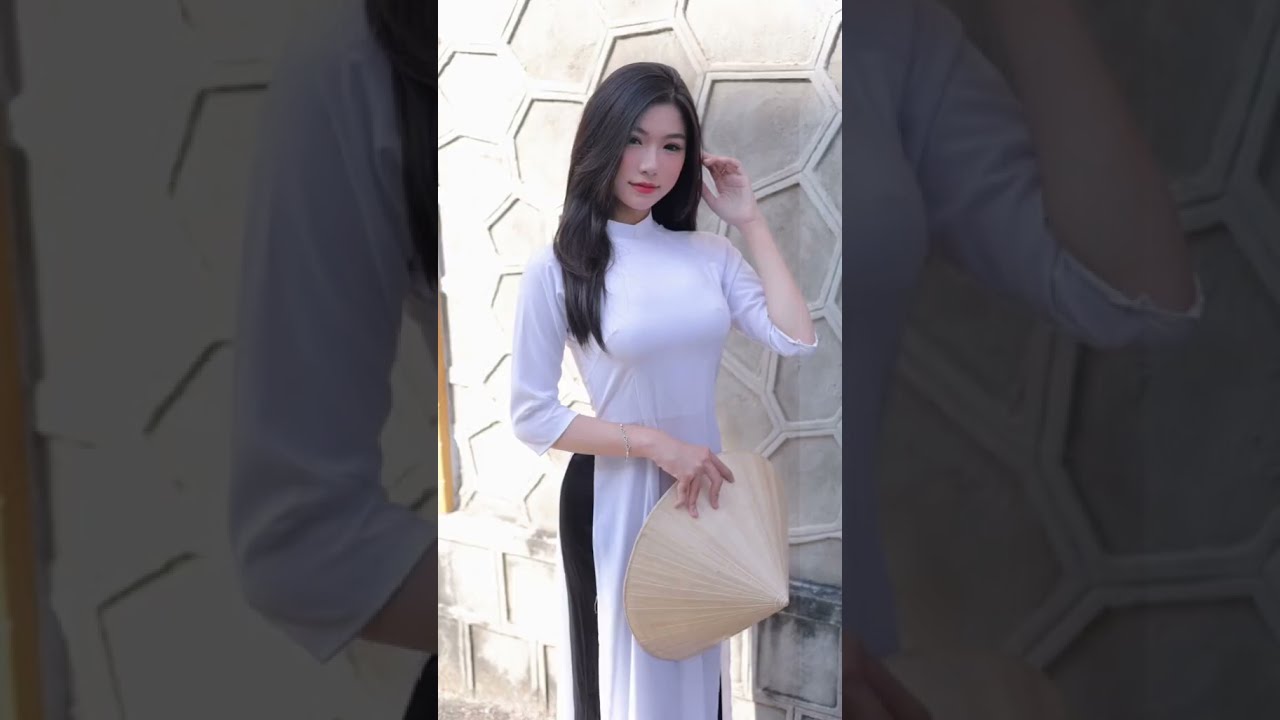The image features a young, attractive Asian woman with long, straight black hair reaching her chest. Her complexion is very pale, and she is adorned with pinkish-red lipstick, subtle blush on her cheeks, and thick black eyebrows. She is dressed in a traditional Vietnamese style gown that is predominantly white with black panels on the sides, and it has slits revealing black pants underneath. In her right hand, she holds a wide, conical straw hat, resembling a traditional Vietnamese farmer’s hat, while her left hand is raised to touch her hair. The background is a textured wall that features a distorted honeycomb-like pattern at the top and transitions into rectangular brick shapes at the bottom. The image has side borders that are enlarged, grayed-out elements derived from the central picture.